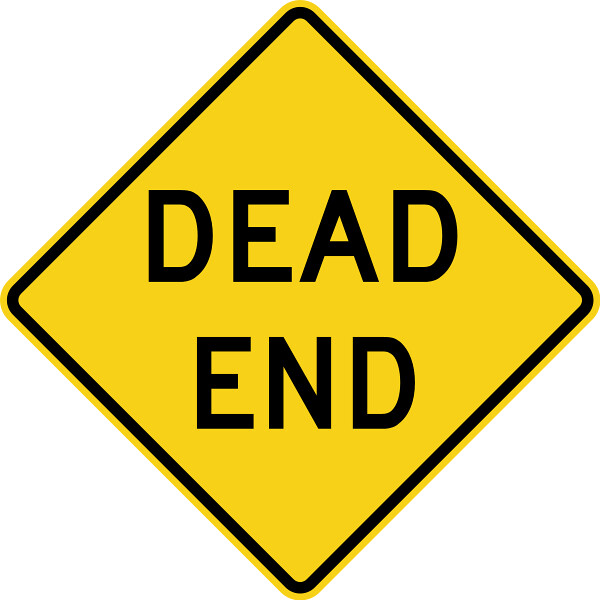The image showcases a prominent dead-end street sign, characterized by its distinctive diamond shape with equal-length sides. This cautionary sign is painted a bright yellow, ensuring high visibility, and is bordered by a thin black line that adds contrast and clarity. Occupying the center of the sign are the bold black letters spelling out "DEAD" atop "END," a message that is immediately noticeable due to its substantial size, covering roughly a third of the sign's surface. The text is designed to be easily readable from a distance, catering to drivers and pedestrians alike. The sign appears against a stark white background, devoid of any context such as a mounting post or surrounding scenery, making the sign the sole focus of the image.